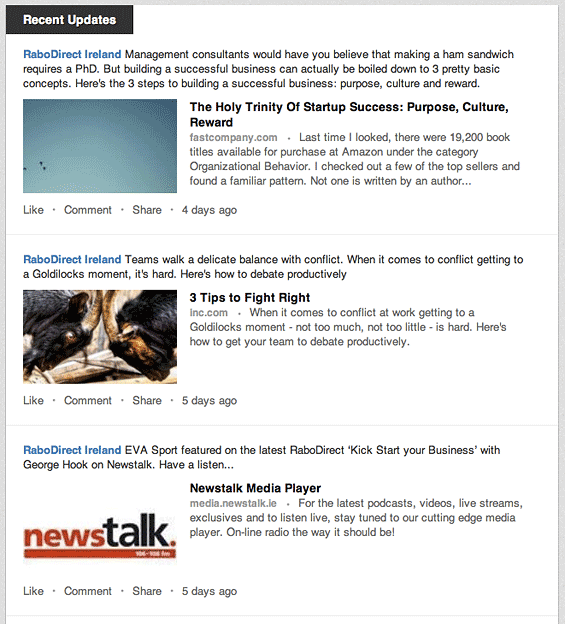The image depicts a news talk-themed media webpage featuring three distinct articles, each offering options to like, comment, or share. The background is white, and the top-left corner features a dark blue or black box with "Recent Updates" in white text. Each article is marked by a blue heading labeled "Rabo Direct Ireland." 

The first article, posted four days ago, is headlined "The Holy Trinity of Startup Success: Purpose, Culture, Reward" in bold black text. It includes a blue thumbnail image that appears to depict the sky. 

The second article, posted five days ago, is titled "Three Tips to Fight Rot" in bold black text and is accompanied by a thumbnail image of two goats or rams headbutting each other.

The third article, also posted five days ago, is titled "News Talk Media Player" in bold black text. Its thumbnail features the News Talk logo, with "News" in red, "Talk" in black, and a red underline beneath "Talk."